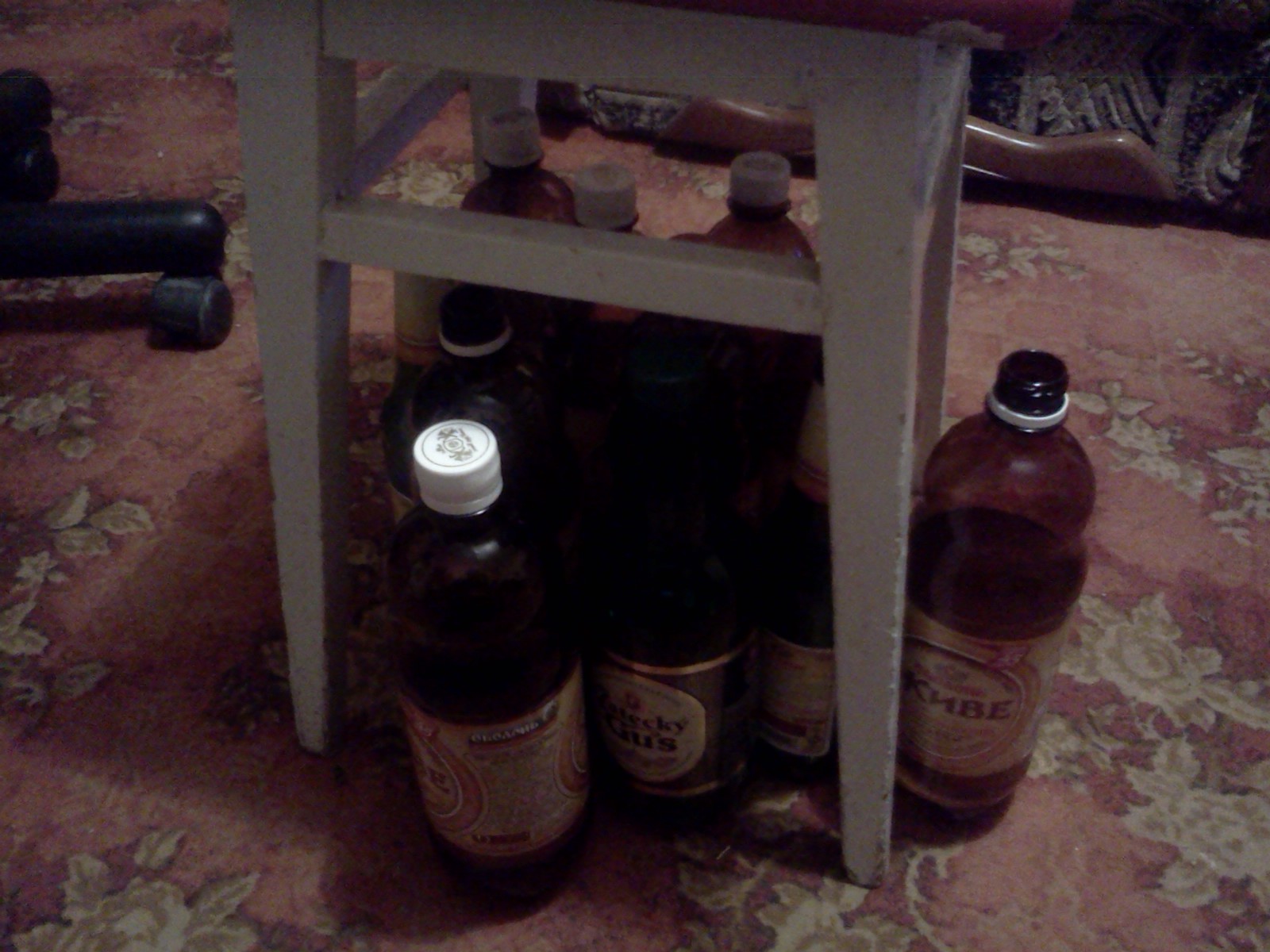The photo depicts an indoor scene with dark lighting, showing a group of about eight brown plastic bottles arranged upright on a pink rug featuring a white floral pattern. Most of the bottles have white plastic caps, although one bottle on the left is missing its cap, revealing a patterned design. The bottles bear similar light brown labels, likely written in a foreign language, possibly Russian. The bottles are situated under a wooden piece of furniture, which could be a table or stool, evidenced by its legs visible in the center. In the top left of the image, the wheels and leg of an office chair are visible, contributing to the room's cluttered appearance.